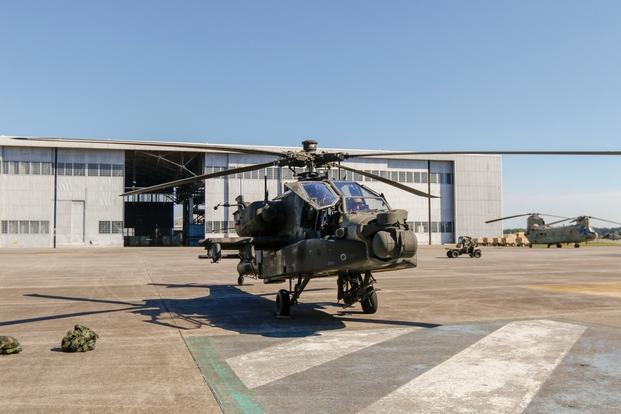A photograph captures a military helicopter stationed on a gray, cement tarmac in front of a large aircraft hangar. The helicopter, painted in an olive green with some camouflage accents, features three wheels and four long blades on its top propeller. One of its front cockpit doors on the left-hand side is open, though it’s difficult to discern if anyone is inside. The ground in front of the helicopter shows a square area with white and aquamarine stripes, albeit dirty and worn. Behind and to the right of the main helicopter, another military helicopter with twin rotors is visible. The hangar, a tall rectangular structure with large metal doors and two sets of windows running along the top and bottom, has its doors open, revealing the expansive interior. The sky is clear blue, and the entire scene is bathed in sunlight, accentuating the muted, rugged colors of the military equipment and the stark, utilitarian environment.